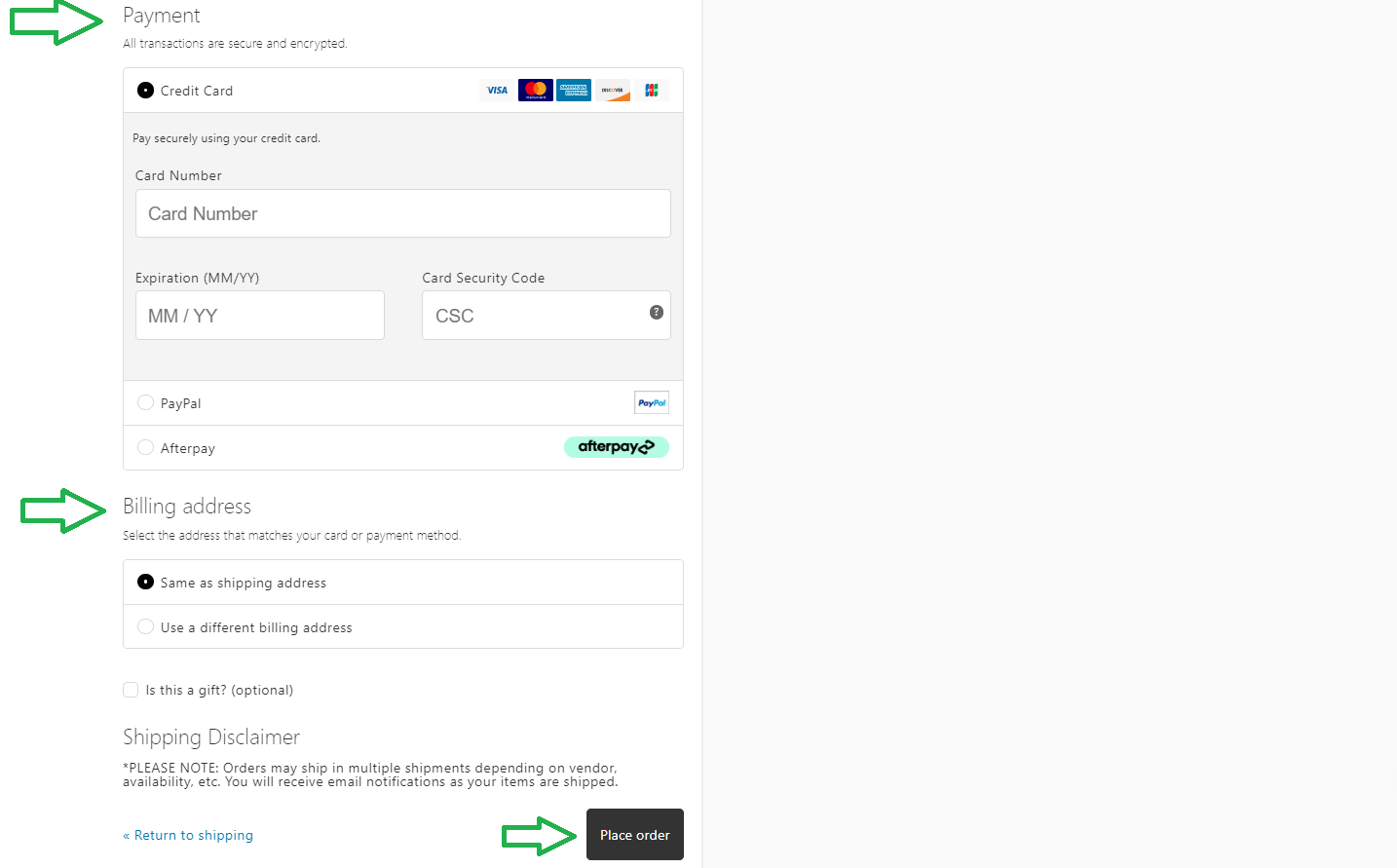**Detailed Caption:**

The image is divided into two sections: a blank gray box on the right side and a detailed illustration of a payment form on the left side. The left side features an image of a pavement area, highlighted with multiple thick green arrows that have white interiors and green borders. The first arrow points to a section labeled "All transactions are secured and encrypted," followed by a list of credit card icons including Visa, MasterCard, and American Express. The phrase "Pay securely using your credit card" is aligned to the left.

Below this, there's a white rectangular box labeled "Credit Card Number," intended for users to enter their credit card information. Following this, the caption "Expiration Date" is accompanied by the format "(MM/YY)" both outside and inside another white rectangular input box. To the right of this section is an area titled "Card Security" with a gray box labeled "CSC" and an adjacent circle containing a question mark, presumably for help or additional information.

Further down, the form mentions "Bill on PayPal" and "Afterpay," followed by a "Billing Address" section highlighted with a green arrow. An option for "Same as Shipping Address" is featured within a black square. There's also a shipping disclaimer present. Finally, at the bottom of the form, there is a black "Place Order" button with an arrow next to it, indicating the final step for completing the transaction.